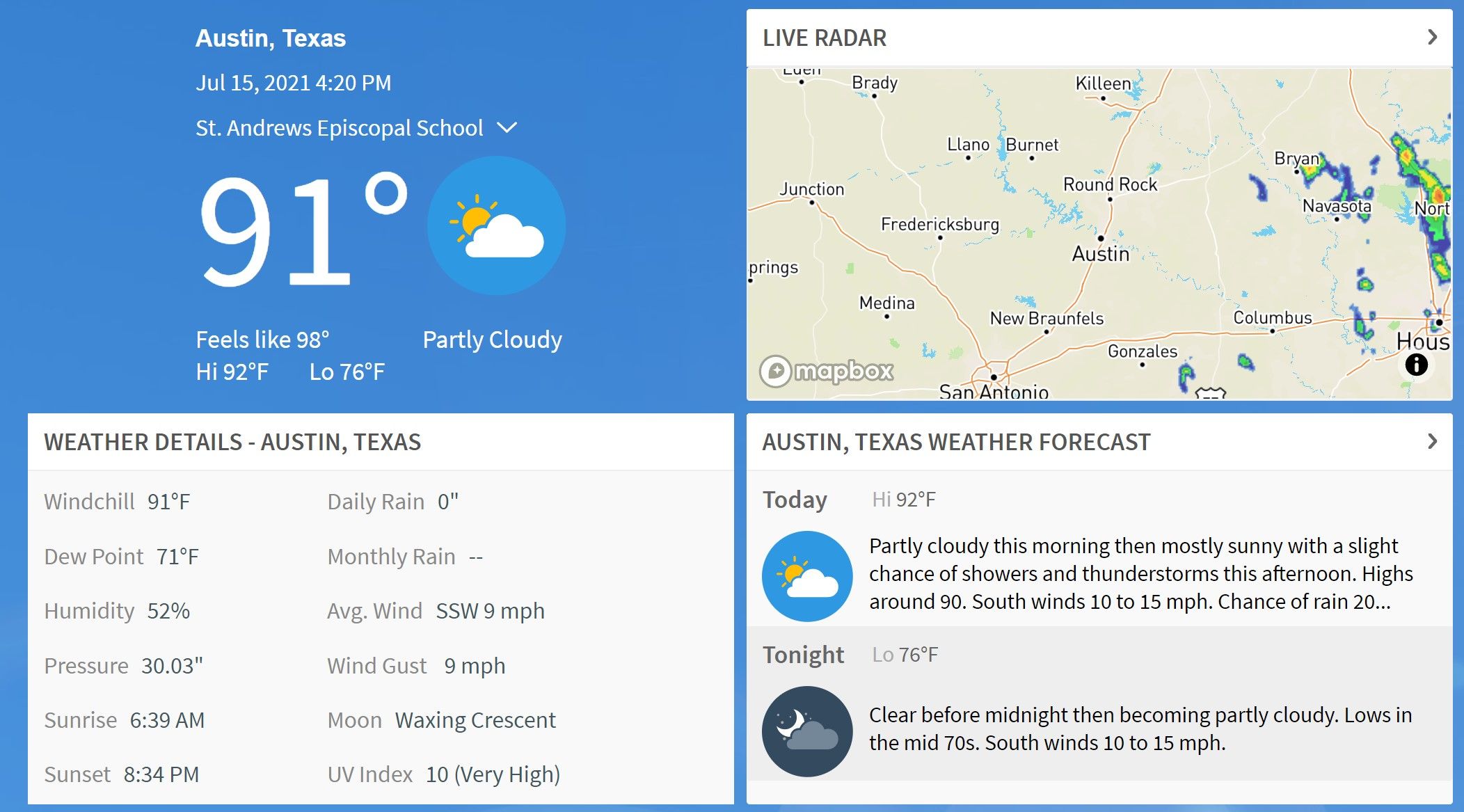The image consists of a rectangular layout divided into four distinct sections, each providing detailed weather information for Austin, Texas. 

In the top left section, a blue panel presents a comprehensive snapshot of the weather for July 15, 2021, at 4:20 PM at St. Andrews Episcopal School. It shows a temperature of 91°F, partly cloudy conditions (illustrated by a small icon), and feels like 98°F. The forecast also indicates a high of 92°F and a low of 76°F.

To the right of this section, the second panel features a live radar map of San Antonio and the surrounding areas, offering a visual representation of current weather conditions in relation to Austin.

The third panel continues with detailed weather metrics for Austin. It includes specifics such as wind chill, daily and monthly rainfall, dew point, humidity, average wind speed, pressure, wind gusts, sunrise and sunset times, moon phase, and the UV index. These details provide a deeper understanding of the local climate beyond the basic temperature overview.

The final section, located at the bottom, gives a detailed weather forecast for Austin. It describes the morning as partly cloudy, transitioning to mostly sunny in the afternoon with a slight chance of showers and thunderstorms. Highs are expected to be around 90°F, with south winds ranging from 10-15 mph and a chance of rain. For the evening, the forecast indicates clear skies before midnight, becoming partly cloudy later on.

This detailed layout offers a thorough and multifaceted view of the weather conditions and forecasts for the specified location and date.